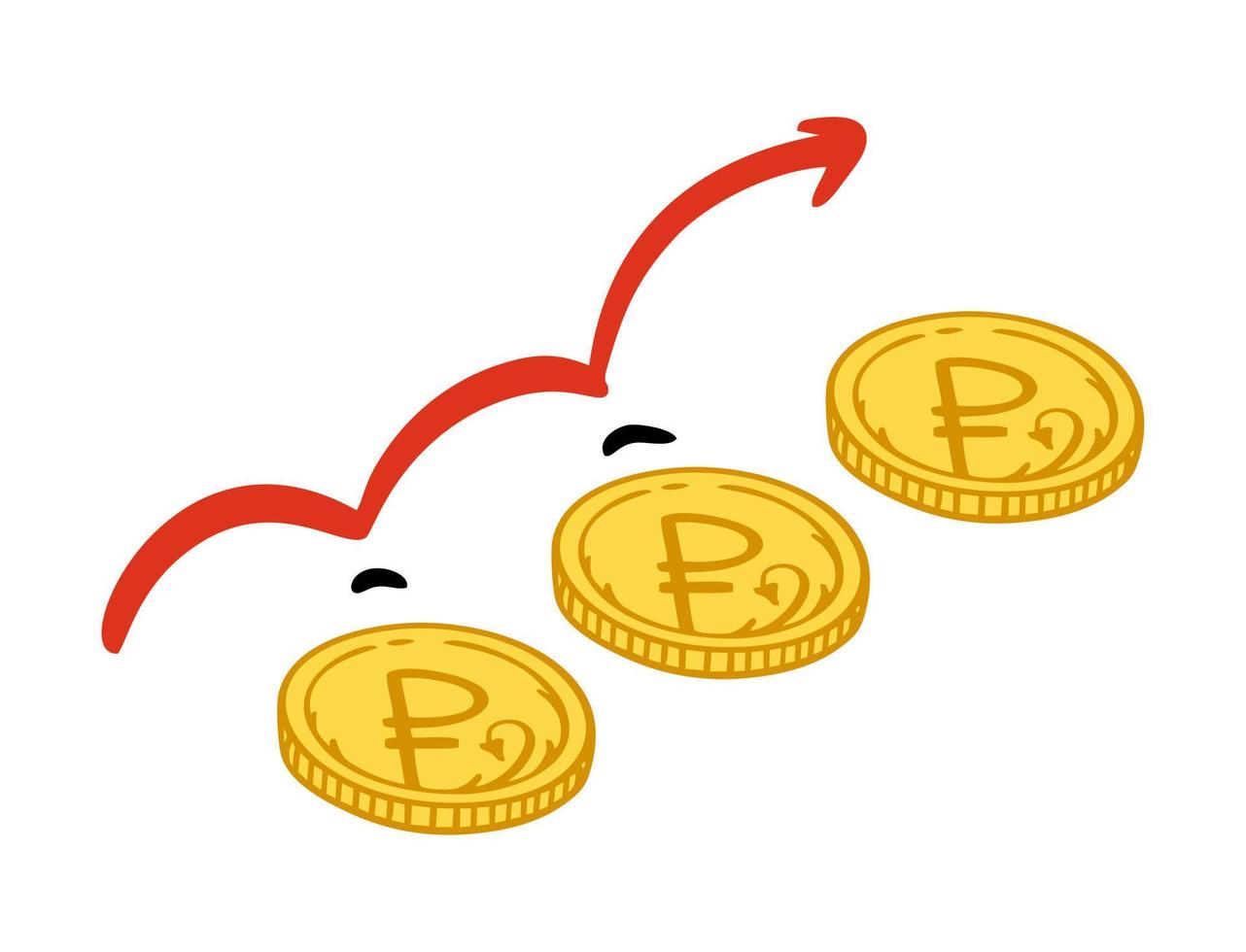This cartoon image depicts a diagonal arrangement of three yellow coins, each featuring a 'P' symbol prominently across the middle and detailed lines along their edges. The coins are evenly spaced, stacked slightly to the top right in a step-like manner. Above them, a dynamic red arrow starts from the left of the first coin, gives the appearance of bouncing off each coin, illustrated by a curved black line, and points over the third coin. The background is stark white, creating a clean and open feel. A subtle black shadow accompanies the coins to the side, adding depth to the vibrant gold, yellow, and red color palette of the illustration.